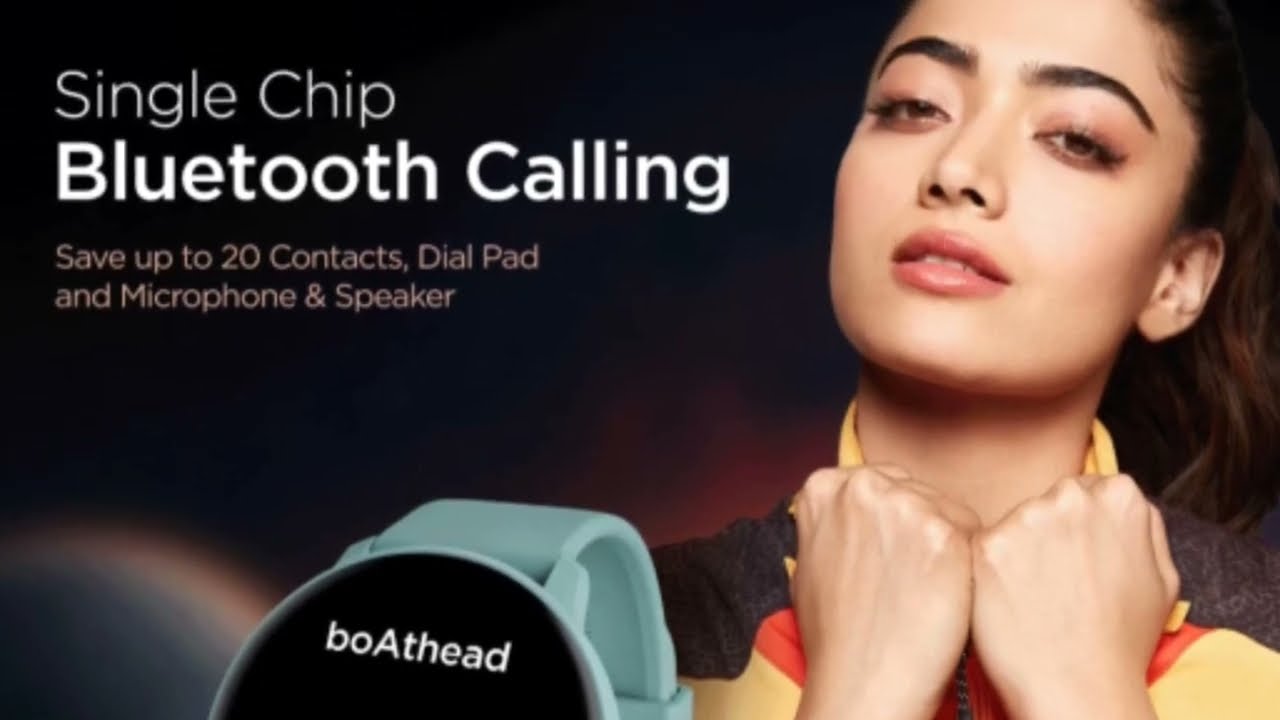This is an advertisement for a Bluetooth smartwatch prominently featuring a woman posing with her fists near her neck. She has pink lipstick, eyeliner, and light-colored eye shadow, with long brown hair flowing down to her shoulders. She is wearing a vibrant shirt with a mix of yellow, black, and red colors, and a black collar. The background is primarily black with a blue spearlike graphic in the bottom left corner.

In the foreground, there's a close-up shot of the smartwatch, which has a turquoise band and a black circular face. The brand name "BOATHEAD" is displayed in white text on the watch face. The advertisement highlights features of the smartwatch in white and purplish text, stating: "Single Chip Bluetooth Calling," "Save up to 20 contacts," "Dial pad," and "Microphone and Speaker."